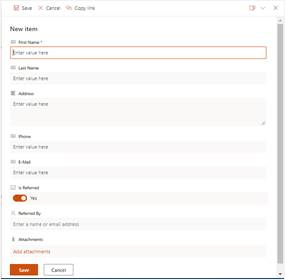This image appears to be a detailed screenshot of a user interface form, possibly from a web application or software. The form is segmented into several categories for user input. At the very top, the black header prominently displays "New Item." Below this header, aligned to the right, there are options to save or copy the form's details, accompanied by an 'X' button in the top right corner, offering the option to cancel or close the form.

Immediately beneath the header, the form begins with a field labeled "First Name," followed by a corresponding input box where users can enter their first names. Directly under this, there is another input field labeled "Last Name," continuing the sequence for personal information entry. The subsequent field is designated for entering an "Airline," though this text is notably challenging to read due to its small size. Following the airline field is a slot for a "Phone" number, allowing users to input their contact number.

Further down, there is an "Email" field for users to input their email addresses. Adjacent to this field is a toggle labeled "Yes," which is currently switched to the right, indicating an active state. At the very bottom of the form, users are given the option to add attachments.

Two prominent buttons for user actions are located at the form's conclusion. The "Save" button is displayed in a bright orange rectangle, while the "Cancel" button is housed in a white rectangle. Overall, the form is presented on a computer screen interface, and it appears to be part of a structured and detailed data entry process.